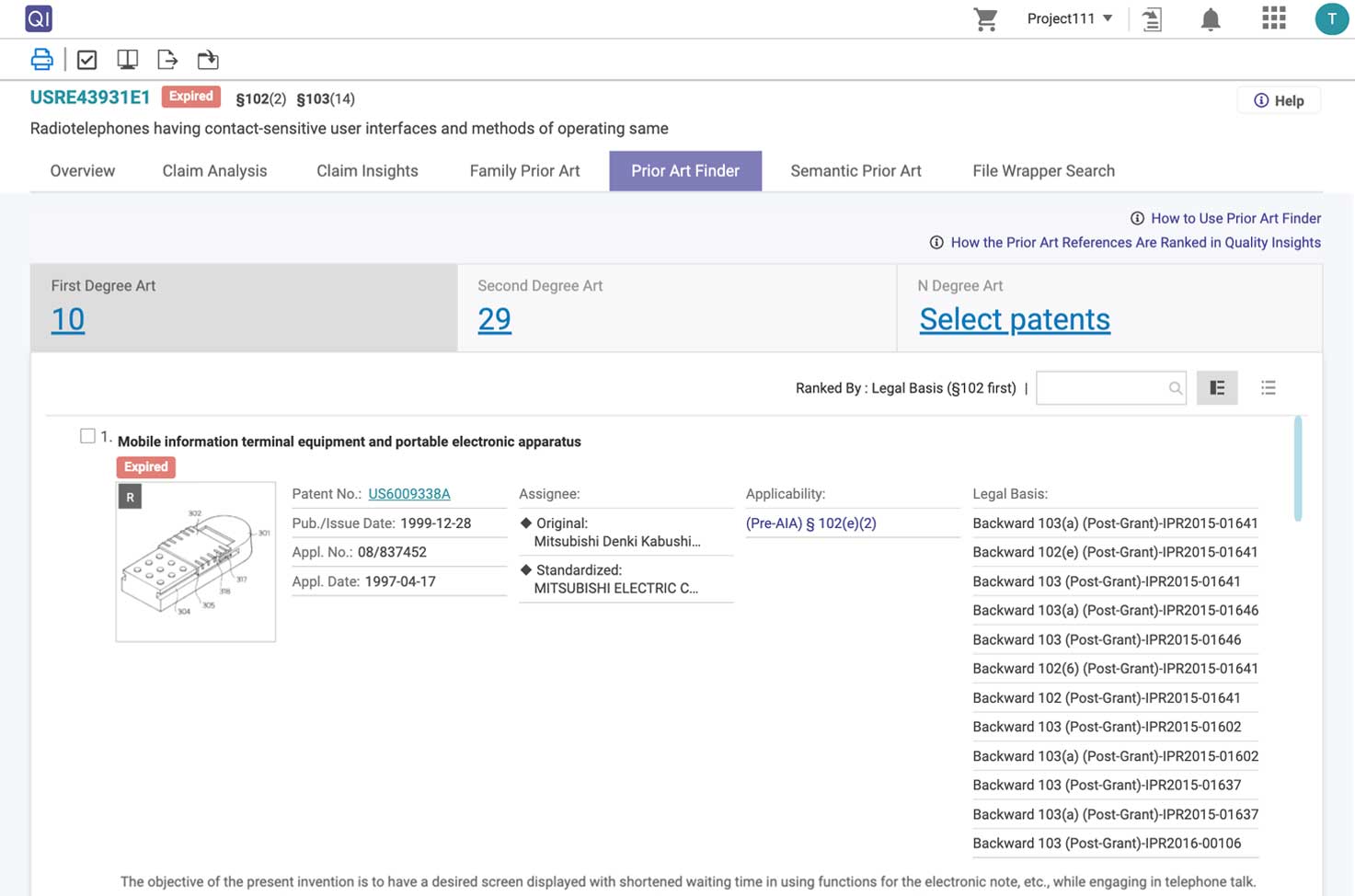The image depicts a website where users can purchase various items. The presence of a shopping cart icon at the top confirms it as a shopping site, and an account indicator suggests that the user is logged in. Notably, a message about something being expired is visible. The site features categories such as radio telephones and sensitive user interfaces, alongside information regarding methods of operation.

Highlighted prominently on the page is an option to explore mobile information, terminal equipment, and portable electronic apparatus, with an emphasis on an expired status. An image of an older telephone is displayed, along with details such as the patent number, assignee, and applicability. Legal basis information is provided, with a specific note that it ranks S-102 first in legal status. On the right side of the page, users can choose from various options, and there is an indication that additional information is available upon scrolling further.